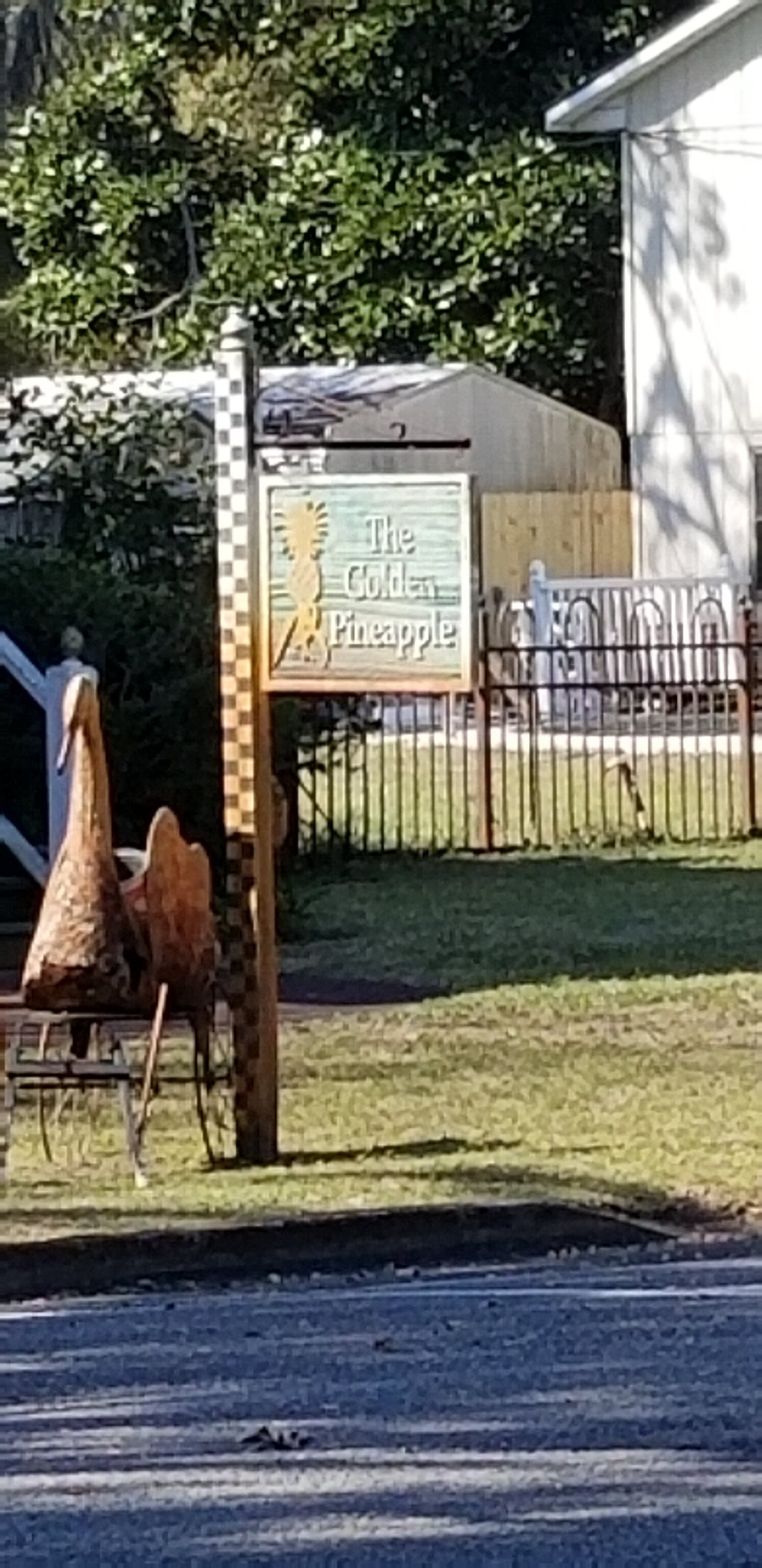The image depicts the entrance to an establishment called "The Golden Pineapple." The focal point of the photo is a signpost adorned with black and white checkered patterns. Extending horizontally from the post is a black metal crossbar, from which hangs a sign crafted from a material that appears to be textured wood or metal. The sign itself has a background of shaded blue hues and displays the words "The Golden Pineapple" in white lettering, along with an illustration of a yellow pineapple.

To the left of this sign is a whimsical, yellow duck or swan-shaped figurine that has a cavity, suggesting it could hold a plant. This figurine is mounted on wheels with metal spokes, giving it a vintage carriage-like appearance. 

The scene is set on a patch of green grass, indicating a well-maintained lawn, with shadows cast by the sun, suggesting a bright day. Beyond the lawn lies a black tar road that glistens slightly under the sunlight. 

In the background, the image captures a metal fence, possibly wrought iron, which stands in front of a white plastic fence. Behind these barriers are various buildings, including a low shed-like structure and a taller white building with a noticeable door or window on its left side. Adding to the scenery are trees that stretch above the rooftops of the buildings, contributing to the picture's outdoor and somewhat residential ambiance.